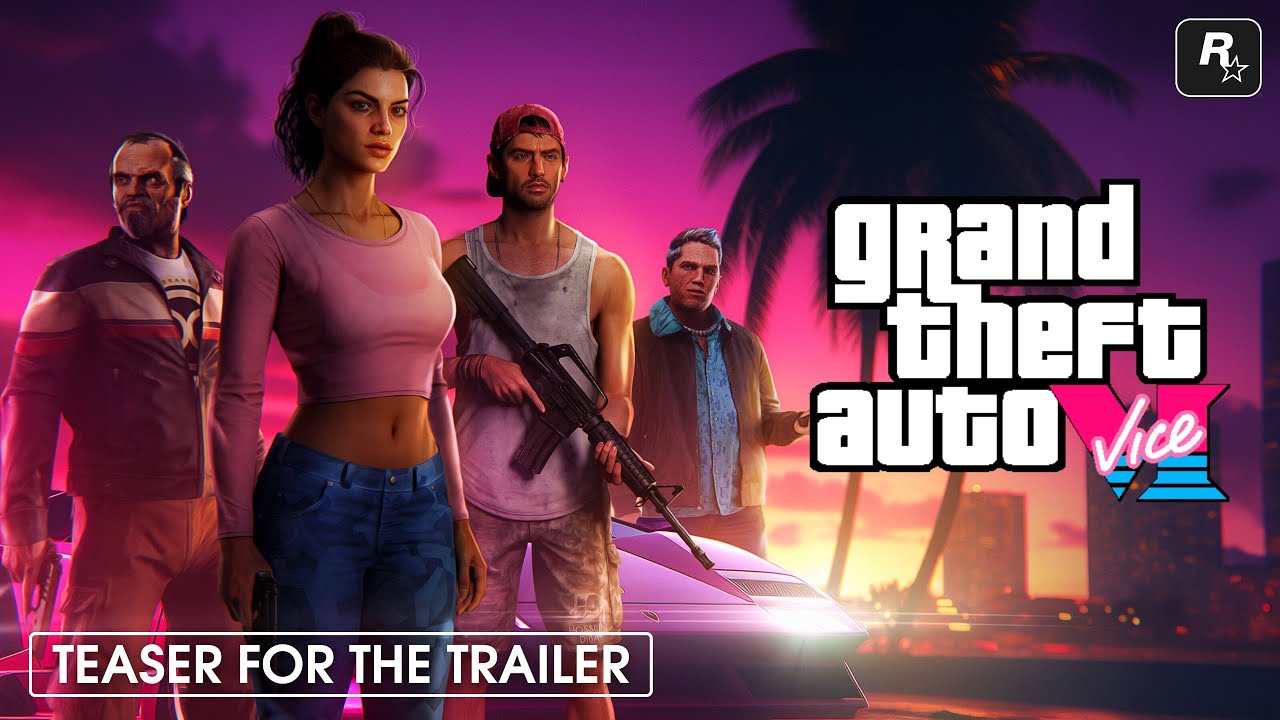This image, presented in landscape orientation, appears to be an advertisement for Grand Theft Auto Vice 6, resembling a potential throwback to Grand Theft Auto Vice City. The right side features the game's title: "Grand Theft Auto" in white letters, with "Vice" in pink, white, and blue hues, all set within a black border. The top right corner displays the Rockstar logo, a distinctive "R" with a star.

Four characters are prominently positioned around a fancy car against an 80s-style cityscape with palm trees. At the forefront is a woman with dark hair, donning a tight pink crop top that reveals her midriff, and blue camo jeans. She holds a pistol by her side. To her left stands a man with receding black-gray hair, sporting a black jacket with a white and red horizontal stripe, a white t-shirt underneath, and tan cargo pants, also holding a pistol. Another male character, to the woman's right, wears a dirty muscle shirt, camo shorts, and a backwards red baseball cap, and carries an automatic weapon. Further to the right is a man in a blue shirt and brown jacket, akin to a character from a previous GTA installment.

The background features vibrant, neon-like 80s lighting, enhancing the nostalgic ambiance. At the bottom left, text in white within a white border reads "teaser for the trailer," indicating the promotional nature of the image.